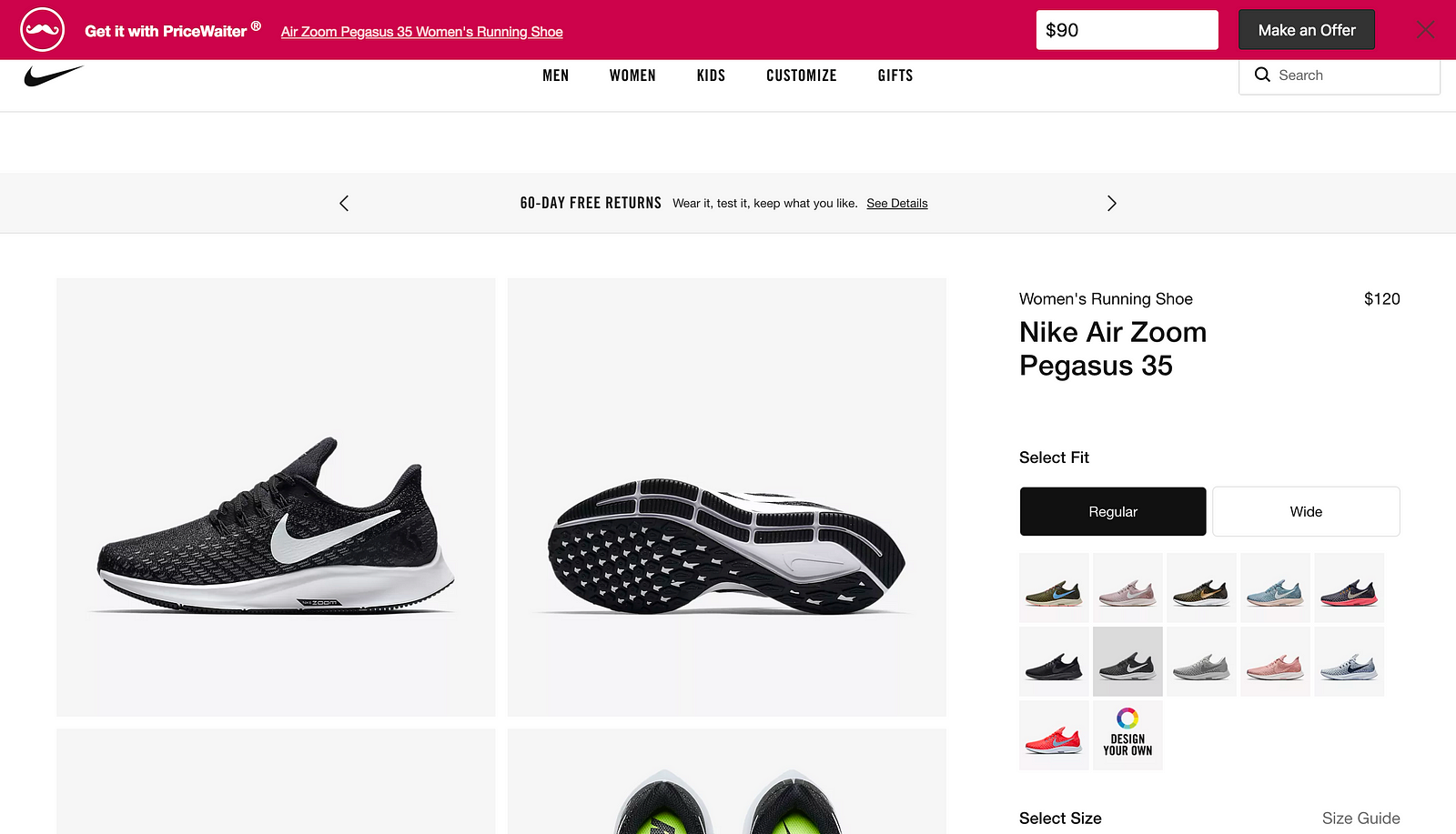This detailed caption elaborately describes a screenshot of the Nike website, specifically focused on the Nike Air Zoom Pegasus 35 women's running shoe.

---

The screenshot depicts the Nike website showcasing the Air Zoom Pegasus 35 women's running shoe. At the top, a red notification bar spans the upper 5% of the screen. On the left side of this bar, there is an icon resembling a handlebar mustache encased in a circle, next to the text "Get it with Price Waiter." Nearby, a search box displays "$90," followed by a black button with white text stating "Make an Offer" and an "X" button.

Below this, the main navigation menu of the Nike website is visible against a white background. It includes a black Nike swoosh logo on the left, followed by category options: Men, Women, Kids, Customize, and Gifts. To the right, there is a search bar marked by a magnifying glass icon.

Further down, a banner highlights Nike's return policy with the text "60-day free returns" and a slogan "Wear it, Keep what you like." This section is flanked by left and right navigation arrows. 

The section featuring the Nike Air Zoom Pegasus 35 shoe includes multiple images on a white background. The first image shows a side view of the shoe angled to the left, featuring a black upper, white lower, and a prominent white Nike swoosh. To the right of it, there's an image of the shoe's sole. Below that, a top view of the shoe is partially visible, slightly cut off.

To the right of the images, descriptive text labels the product as the "Nike Air Zoom Pegasus 35 Women's Running Shoe" priced at $120. Options for selecting fit (Regular and Wide) are available, alongside a variety of color choices displayed further down.